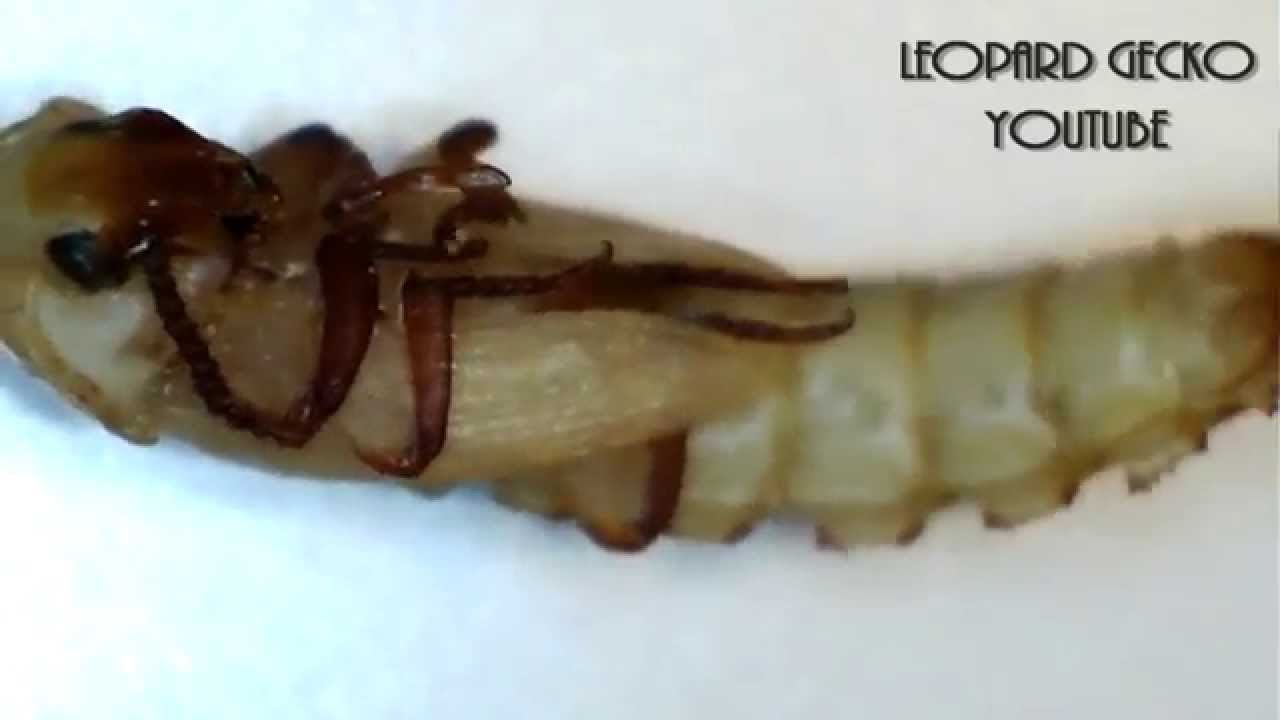This is a detailed close-up photograph of an arthropod larva or a bug-like creature, potentially in its larval stage, lying on its back. The image features text in the top right corner reading "LEOPARD GECKO" in black capital letters with "YouTube" written below it. The background transitions from a grayish-white color on the right side to a bluish-white hue on the left. The creature, which may be a type of segmented worm like a mealworm or a cricket, is showcased horizontally with its head on the left and tail on the right. It exhibits a beige or yellowish-brown segmented body, adorned with dark brown legs that curve inward, and blackish-brown eyes. The overall image highlights the intricate details of the larva's body sections and limb structures, despite the slight translucency and indistinct clarity of the photo.